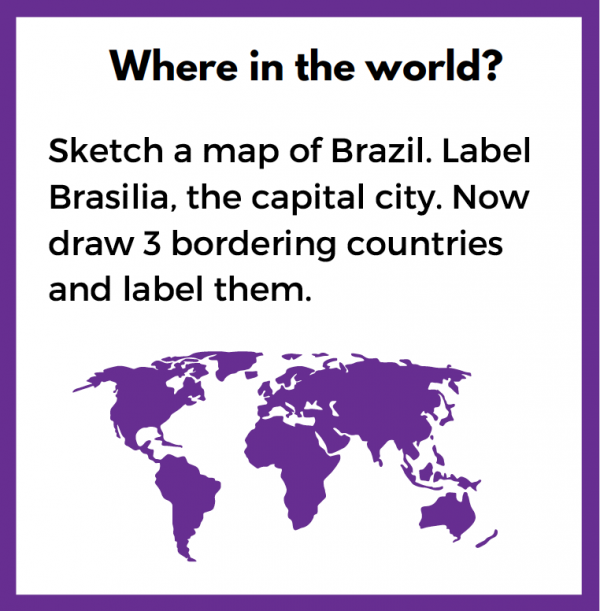A detailed assignment worksheet is depicted in the image, presented within a white square bordered by a purple trim. The purple edging frames the worksheet elegantly, drawing attention to its central contents. At the top of the worksheet, bold and centered text reads, "Where in the World?" This heading leads into the primary task instructions, which are meticulously printed below: "Sketch a map of Brazil. Label Brasília, the capital city. Now, draw three bordering countries and label them."

The bottom part of the worksheet features an outlined sketch of all seven continents displayed in a flat, Mercator projection style. This world map is intended as a base for the student's work. The instructions imply that students are to use this global map to sketch Brazil's map, marking Brasília and identifying three of its neighboring countries. Although the worksheet hints at a digital format, indicated by its clean and precise layout, there is no visible "submit" button or any other digital submission instructions, suggesting it might also be designed for physical print-out and manual completion.

Overall, this structured assignment challenges students to apply their geographical knowledge of Brazil within the global context provided by the world map sketch.